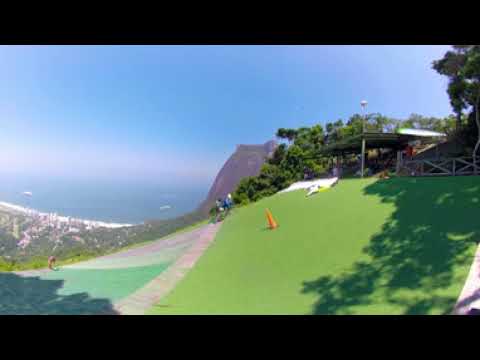The image captures a lush, green hillside dotted with an orange traffic cone, which serves as a marker amid the well-maintained grass that almost resembles astroturf. The grassy hill is populated with a few people hiking up the slope, and it gently descends towards a picturesque ocean in the distance. The backdrop features a panoramic mountain range with a volcano-like peak, reminiscent of an exotic locale like Hawaii. The turquoise sky above is clear yet slightly misty, casting shadows of the scattered trees onto the landscape. A brown wooden fence separates the grassy area from a concrete bike trail, which meanders through the scene. To the left, a solitary figure is bending over, and at the top of the hill, a pavilion stands against the backdrop of crystal-clear, teal ocean waves crashing onto the sandy shore. The sun shines brightly, enhancing the vibrant colors and bringing the entire scenic vista to life.